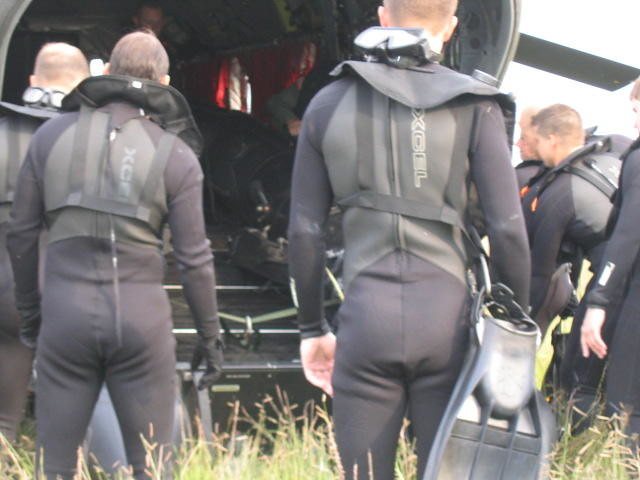The image portrays a group of young men, likely in their 20s, all clad in dark gray wetsuits accented with lighter gray highlights. Each has a pair of goggles around their neck, facing backwards, and holds flippers or instrument bags in their hands. They are gathered in a field of knee to mid-thigh high grass, facing away from the camera, towards a black and gray helicopter. The helicopter, positioned on the left side of the image, features a red and white highlighted rear ramp that is lowered, suggesting they are about to board. A stationary propeller blade is visible against the gray-white sky in the upper right corner. The men, possibly military personnel like Navy SEALs, appear clean-shaven and are outfitted with life vests. The closest individual in the bottom right corner stands out more, prominently displaying his flippers attached to a carabiner.